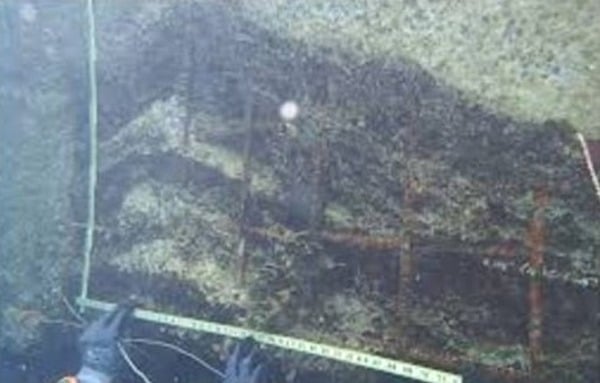This is a color photograph depicting a dimly lit, hazy scene with dark, muted, and murky colors. The image appears blurry and primarily features shades of green and brown. Near the bottom of the photograph, a pair of hands wearing blue or dark gloves are clearly visible, holding a large measuring stick or yardstick. One measuring stick is being held horizontally, while another extends vertically up the image, indicating a measuring task is underway. The background possibly shows dense vegetation, including trees, though it is somewhat indistinct. There are also elements that suggest the scene might be underwater, with rusted bars and green algae visible, contributing to the overall unclear and dark appearance of the photograph. Illumination seems to come from a single light source, possibly the camera flash, highlighting the gloves and measuring instruments while leaving much of the scenery in shadow.